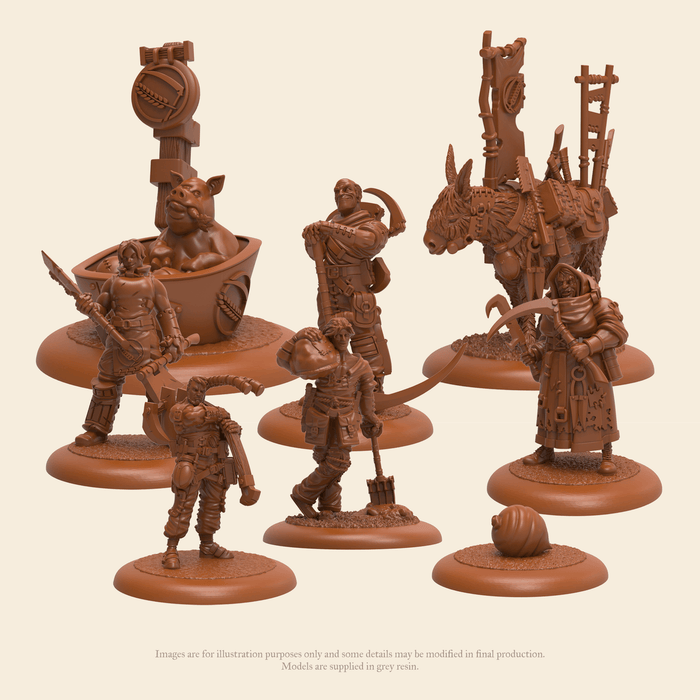In the center of the image, which features a beige background and accompanying text at the bottom stating "images are for illustration purposes only, and some details may be modified in final production. Models are supplied in gray resin," there are several intricately designed miniature figures. These miniatures are likely intended for a tabletop game and are depicted on round bases. 

Starting from the top left, there's a whimsical figure of a pig sitting in a bathtub, depicted with a carrot in its mouth and large, expressive ears. Behind the pig, a tall sign adorned with symbols and a flower icon adds to the fantasy theme. At the top right stands a sturdy mule or donkey, burdened with a variety of tools on its back, lending a utilitarian charm to the set.

Moving to the bottom right, there is a peculiar, acorn-shaped miniature figure, which might represent a vegetable character, adding a quirky element to the collection. Adjacent to it, a smaller figure appears to be sweeping the ground with a broom, indicating a more mundane yet essential role in the fantasy world.

Among the various figures, prominent warriors stand out: one is depicted as a steadfast warrior holding a sword and shield with intricate armor and a helmet, while another armored figure holds what seems to be a staff or banner adorned with timbals. All of these miniature sculptures are designed with great attention to detail, capturing the essence of their fantasy roles and emitting a whimsical, adventurous aura.